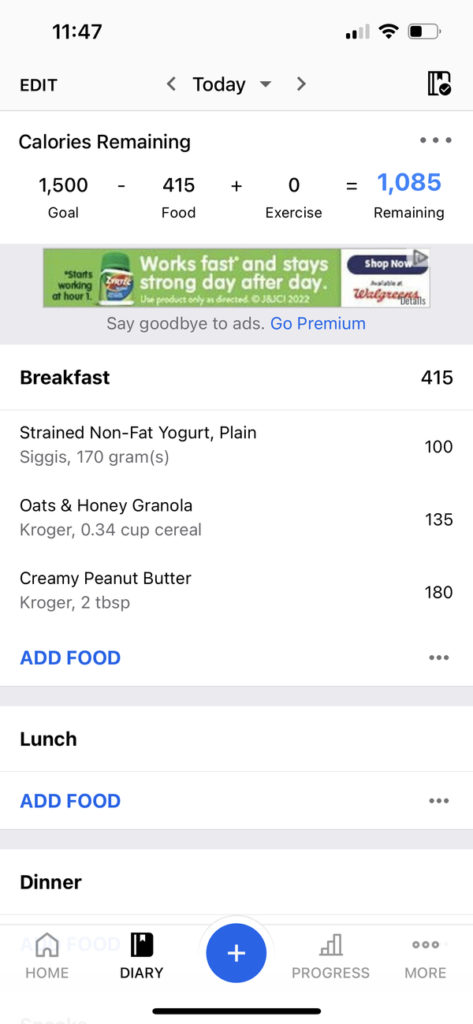The image appears to be a screenshot of a health tracking app on a smartphone with a light rays background. In the top left corner, it displays the time as "11:47" in black text, with the word "EDIT" in all capital letters below it. In the middle of the screen, it says "TODAY". The battery indicator is approximately 40% full and black in color, indicating the battery level. The Wi-Fi icon shows full black bars, indicating strong Wi-Fi reception, while the cellular signal shows two out of four bars in black, indicating moderate reception.

A thin gray line runs across the screen, below which is a section that reads "CALORIES REMAINING" in black. This section details the calorie count as "1,500 goal - 415 food + 0 exercise" and calculates the remaining calories to be "1,085" in blue. Below this, in black again, it states "REMAINING".

There is a gray rectangle containing a green sub-rectangle within it, which features the text "WORKS FAST AND STAYS STRONG DAY AFTER DAY" in white, suggesting an advertisement for allergy medicine likely named Xertex. Beneath this, green text reads "START WORKING AT HOUR 1". Additional text in gray says "SAY GOODBYE TO ADS" with an option in blue to "GO PREMIUM".

Returning to a white background, the app lists breakfast details with "BREAKFAST, 415" in black. The items logged for breakfast include "STRAIN, NON-FAT YOGURT, PLAIN" with 100 calories, "CIGGY'S, 170 grams" (possibly a typo or shorthand for something specific), "OATS AND HONEY, GRANOLA, 135", "KROGER, 0.34 CUP CEREAL", and "CREAMY PEANUT BUTTER, 180" from Kroger, specified as "2 TBSP".